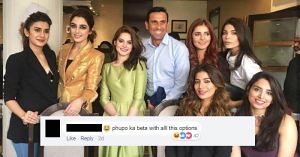In this detailed photograph, we see a formally posed group of eight people, consisting of seven women and one man. The central figures appear to be the focus of the image—a man dressed in a light blue button-up collared shirt, standing alongside a woman in an elegant golden dress. 

The other individuals are equally stylish and poised. To the left, a woman donning a tailored black blazer over a black blouse and blue jeans stands confidently with her dark hair pulled back. Beside her, another woman is clad in a striking gold-colored blazer with a black top underneath, her dark hair similarly pulled back. The next woman dazzles in a shiny green dress and has shoulder-length brown hair.

To the right of the man, another woman with long, dark hair quietly blends into the background as her outfit is not clearly visible. Next to her, a woman in a white top has long, dark hair flowing down her back. Continuing to the right, a woman dressed in black with feathered long dark hair stands gracefully. Finally, the last woman in the lineup wears a dark-colored sleeveless top, her long dark hair cascading down her chest.

All of them are smiling and looking directly at the camera, radiating warmth and unity. The image features an overlay resembling a Facebook comment, which is written in a different language and appears quite blurry, with visible reactions and little emojis indicating likes and other responses.